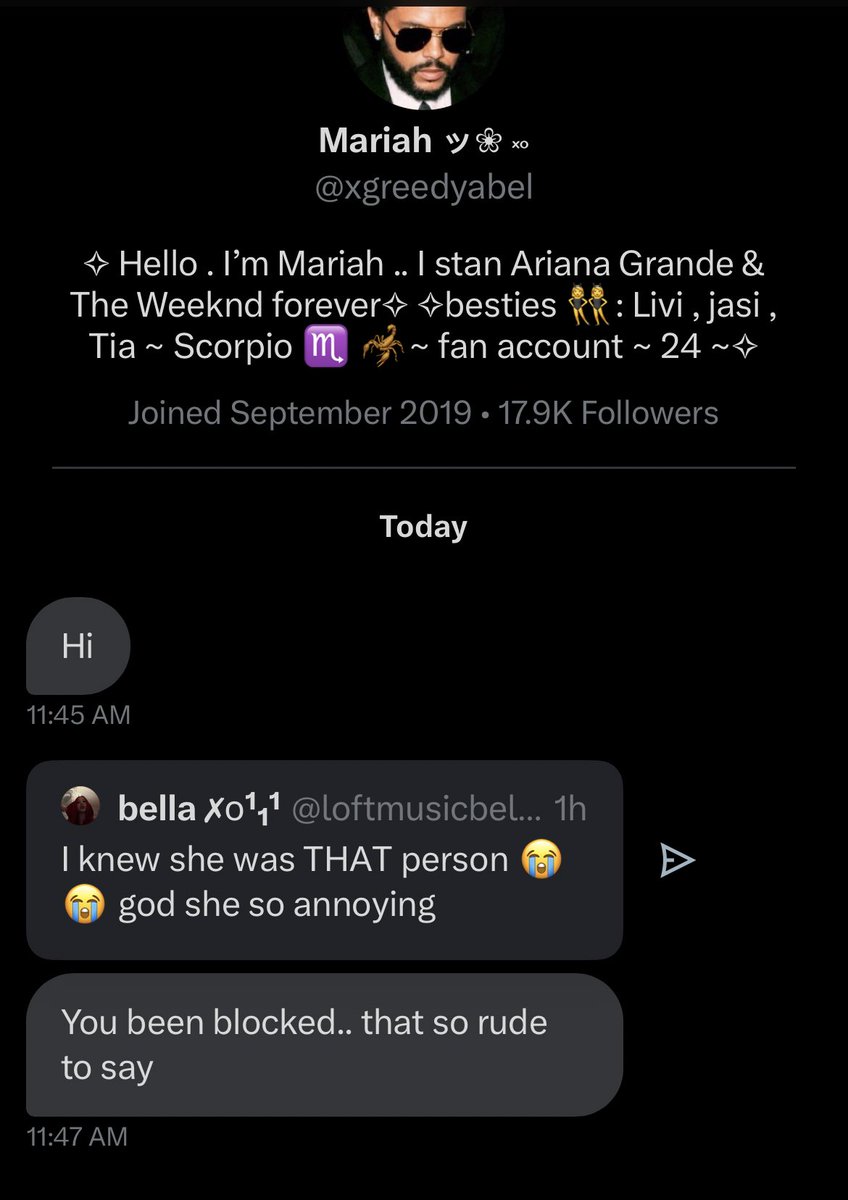This image appears to be a screenshot taken from a mobile device, either a phone or a tablet. At the top of the screen, there is a profile picture of a man wearing sunglasses and sporting a beard. Directly below this image, the profile information reads: "Mariah, 🌸 - @ex_greedy_Abel." The profile description states: "Hello, I'm Mariah. I stan Ariana Grande and The Weeknd forever. Besties: Libby, Jazzy, Tia. Scorpio. Fan account. 💕" The profile indicates Mariah joined in September 2019 and has amassed 179,000 followers.

The lower portion of the screenshot captures what appears to be a message board or chat conversation. At 11:45 a.m., user BellaXO111 (@locked_music_bell) stated, "I knew she was that person," accompanied by two crying face emojis. Shortly afterward, at 11:47 a.m., another message highlighted reads, "God, she's annoying. You've been blocked, that's so rude to say."